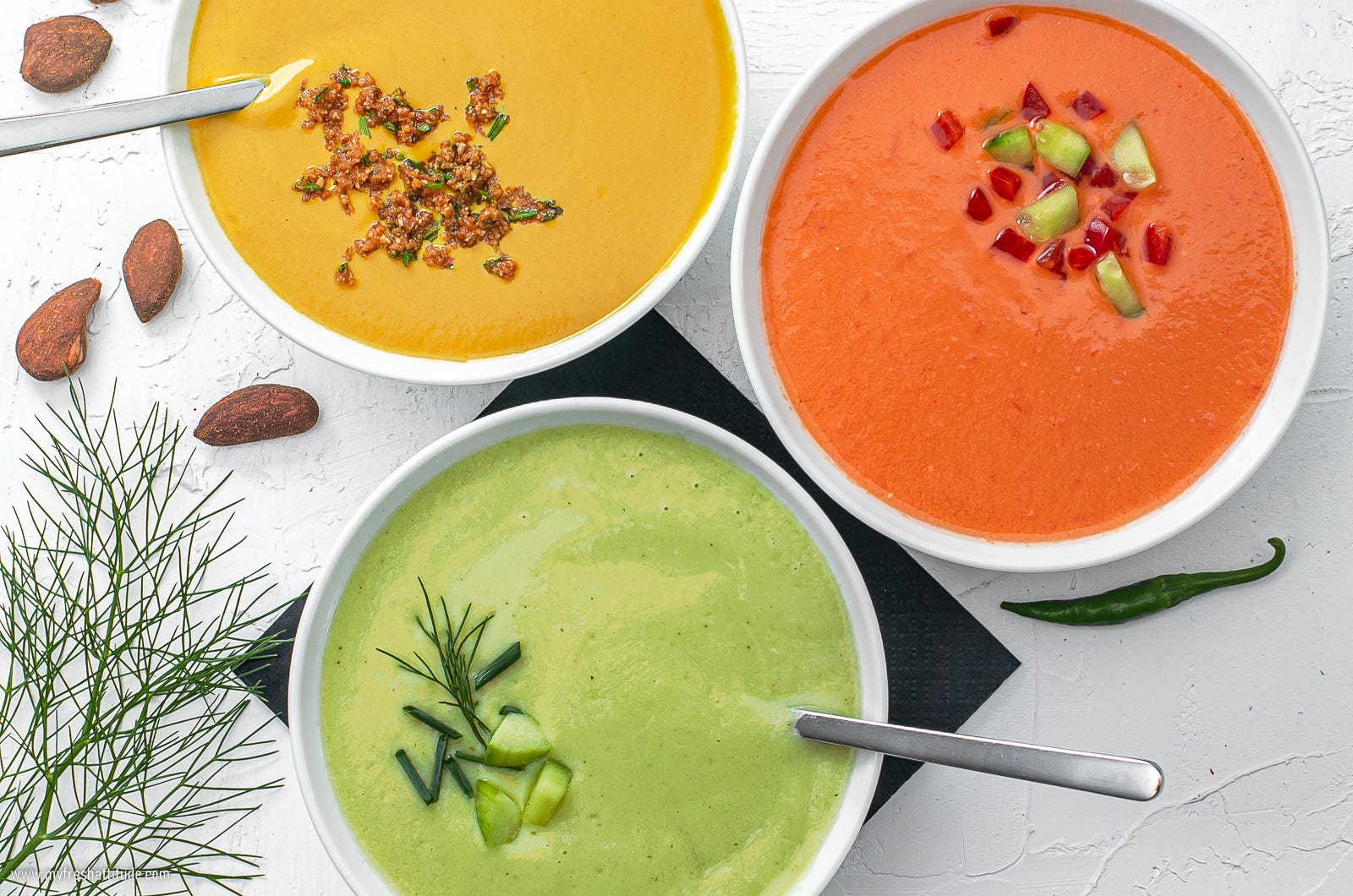This image captures a clean, minimalist setting viewed from directly above, featuring three white bowls of soup arranged on a textured white surface that has visible cracks and subtle 3D-like lines. The surface is accented by a few elements: to the left, there are four small brown rocks or seasoned nuts, and thin green spiny herbs growing up from the bottom left corner. On the bottom right, a small green pepper is partially visible.

The three bowls of soup are distinct and visually appealing. The bowl at the bottom contains a green soup, garnished with chunks of either avocado or cucumber and topped with the same green herbs seen in the bottom left corner. A metallic spoon with only its handle visible rests on this bowl. The bowl on the top left features a creamy butternut squash-colored soup, adorned with what appear to be bacon bits and chives, and also has a spoon whose handle extends out. Finally, the bowl on the top right holds a thick orange soup with green and red chunks, possibly tomato-based, accompanied by a green pepper positioned underneath it.